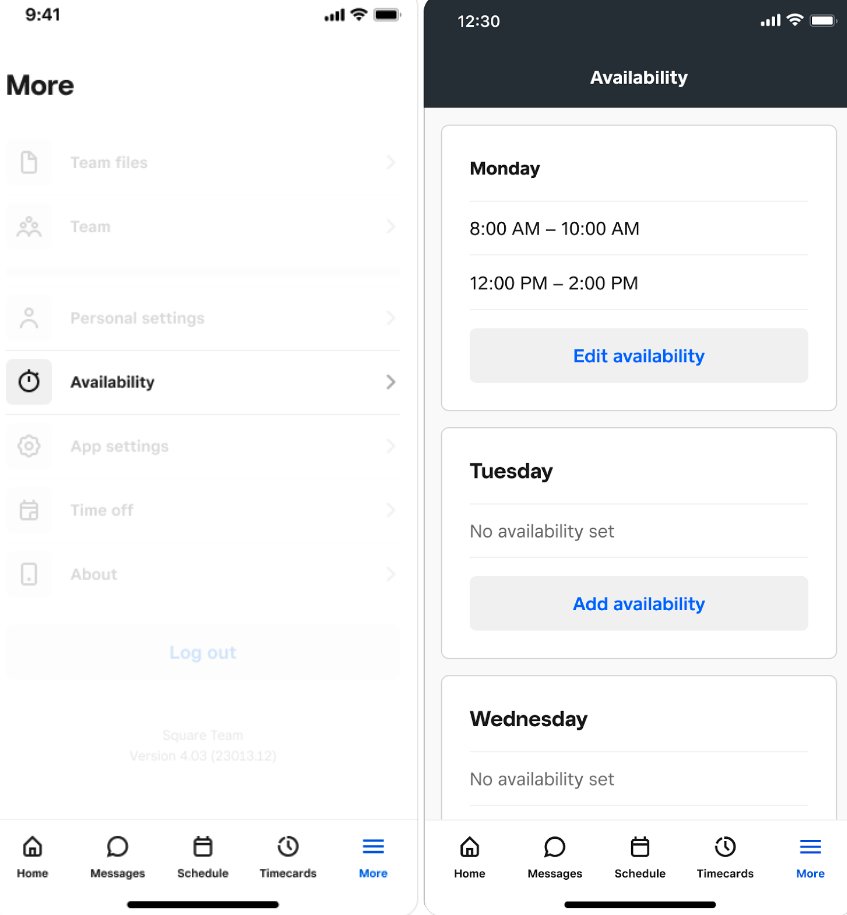The image is divided into two distinct sections. 

On the left side, the layout resembles a cell phone screen with a white background. At the top, the display shows the time as 9:41, with a full horizontal battery icon filled in black. Below the time, the word "more" appears in black text. Underneath this, there are options labeled "Team Files," "Team and Personal Settings," followed by a small gray square featuring a clock icon and the word "Availability" beside it. Further options include "App Settings," "Time Off," and "About," with "Log Out" shown in very light blue text at the bottom.

On the right side, the top background is black, displaying the time as 12:30, with the word "Availability" in white. The area is subdivided into sections:
- The first section shows "Monday," with time slots listed as "8 a.m. - 10 a.m." and "12 p.m. - 2 p.m." Below these time slots, a long blue rectangle states "Edit Availability."
- The next section indicates "Tuesday," with the text "No availability set" and an option "Add Availability" in blue.
- The final section lists "Wednesday," also with "No availability set."

At the bottom of the screen, buttons labeled "Home," "Messages," "Schedule," and "Time Cards" are displayed. The word "More" appears in blue.